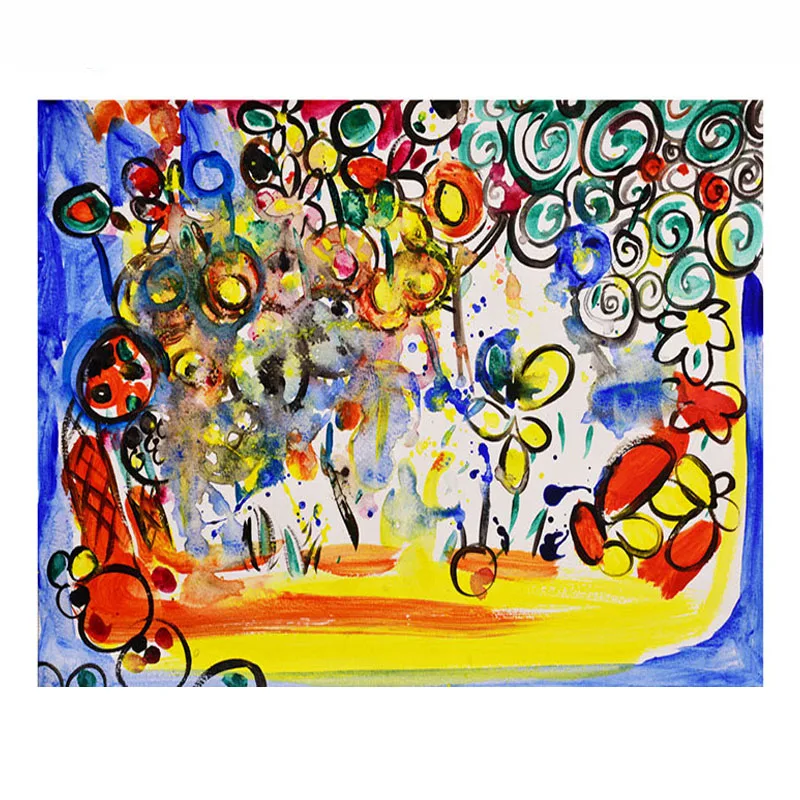This modern abstract impressionist painting depicts a vibrant and colorful scene that combines elements of both representational and non-representational art. Various spirals and circular shapes in vivid hues of greens, reds, oranges, yellows, and blues dominate the canvas, likely representing flowers and other natural forms. These colors blend into a dynamic pool of shifting orange, yellow, and blue at the bottom of the image. A prominent garden of flower-like shapes on the left side, characterized by red outer circles and yellow centers, adds to the lively composition. The left side also features a crisscrossed pattern suggesting a figure, interpreted as a little girl, with an orange circular head, black bangs, and a round body. The center left has a rough patch where the paint seems to have been scraped, creating a textured mix of colors. Meanwhile, the bottom right is filled with additional flower shapes in shades of orange and yellow. Black outlines and smudges interspersed throughout the painting add depth and contrast to this captivatingly colorful piece.